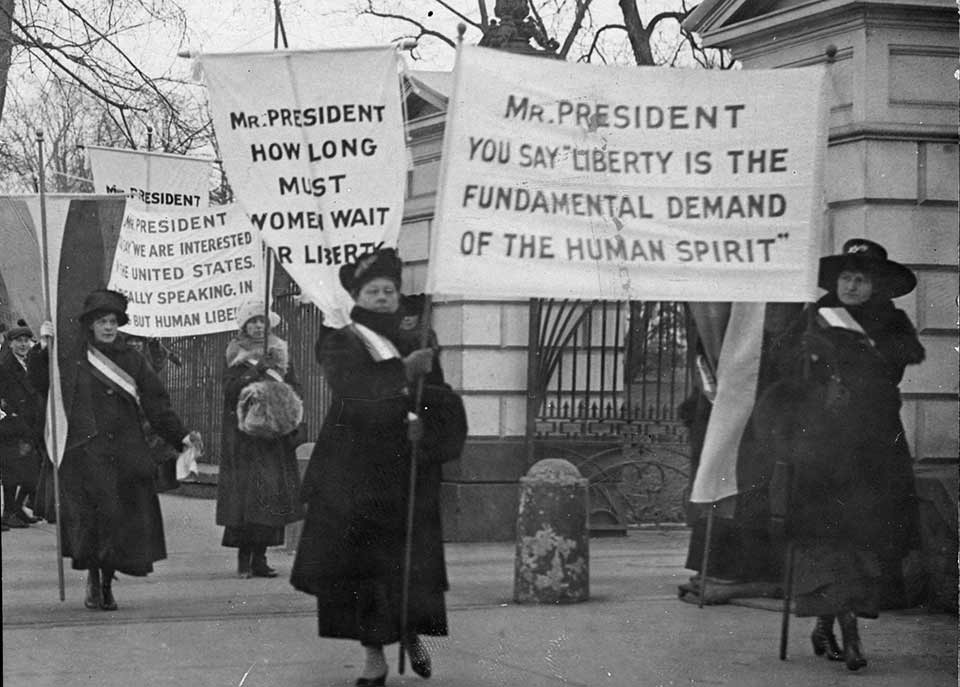The image depicts an old black and white scene of women protesters, likely from the women's suffrage movement, gathered outside a significant building, possibly the White House, inferred from the large white pillars and metal gates in the background. Most women are dressed in long black dresses and black hats, each wearing a distinctive sash over one shoulder, characterized by a white center flanked by two darker stripes. In the foreground, a woman on the left holds a flag with the same sash design. The protesters carry banners and signs in black and white, with one prominent sign reading, "Mr. President, you say liberty is the fundamental demand of the human spirit." The messages on the signs advocate for women's liberties and human rights.